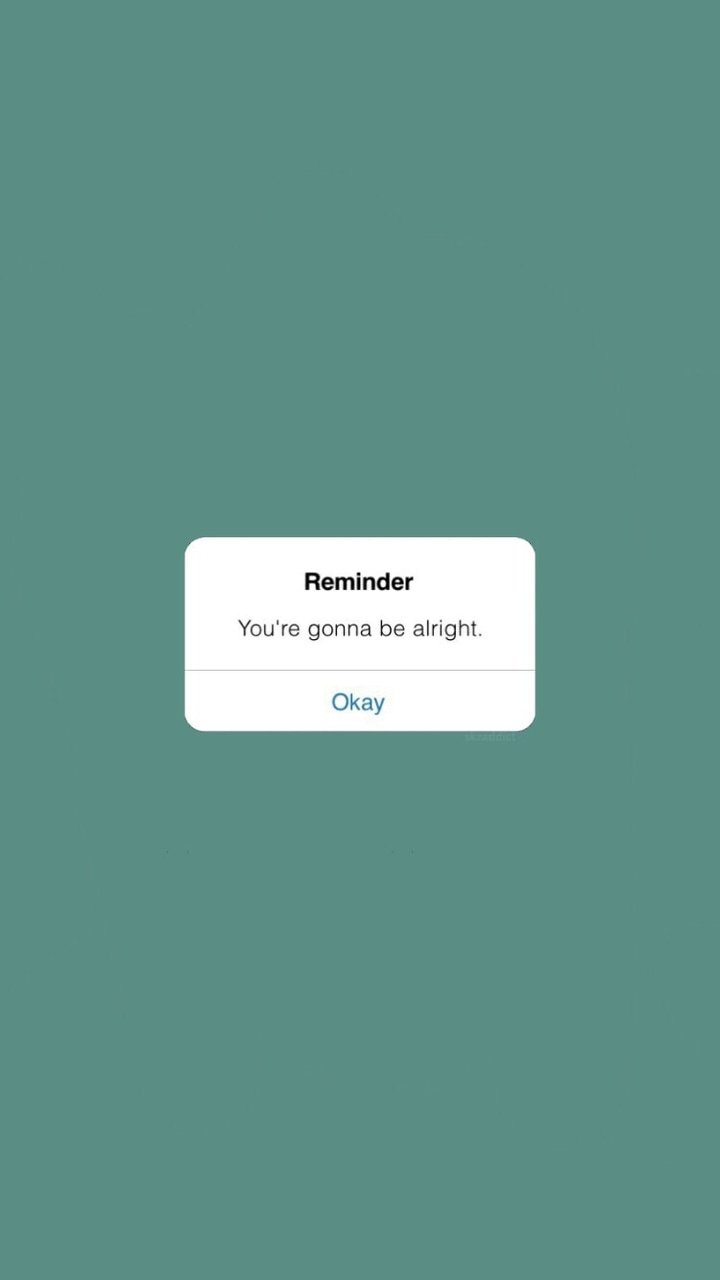The image features a minimalist notification pop-up against a solid blue background. The notification is enclosed within a white rectangular box with all four corners rounded off, providing a soft, approachable look. At the top of the box is the word "Reminder" in black, bold font with the "R" capitalized. Beneath that, in a regular black font, is the reassuring message: "You're going to be alright." The "Y" in "You're" is capitalized, and the sentence concludes with a period, adding a touch of finality and assurance. A thin grey or black line separates this message from a blue button at the bottom of the notification box. The button contains the word "Okay," with the "O" capitalized, inviting the user to acknowledge and dismiss the reminder. Overall, the simple yet carefully designed elements convey a sense of calm and reassurance.